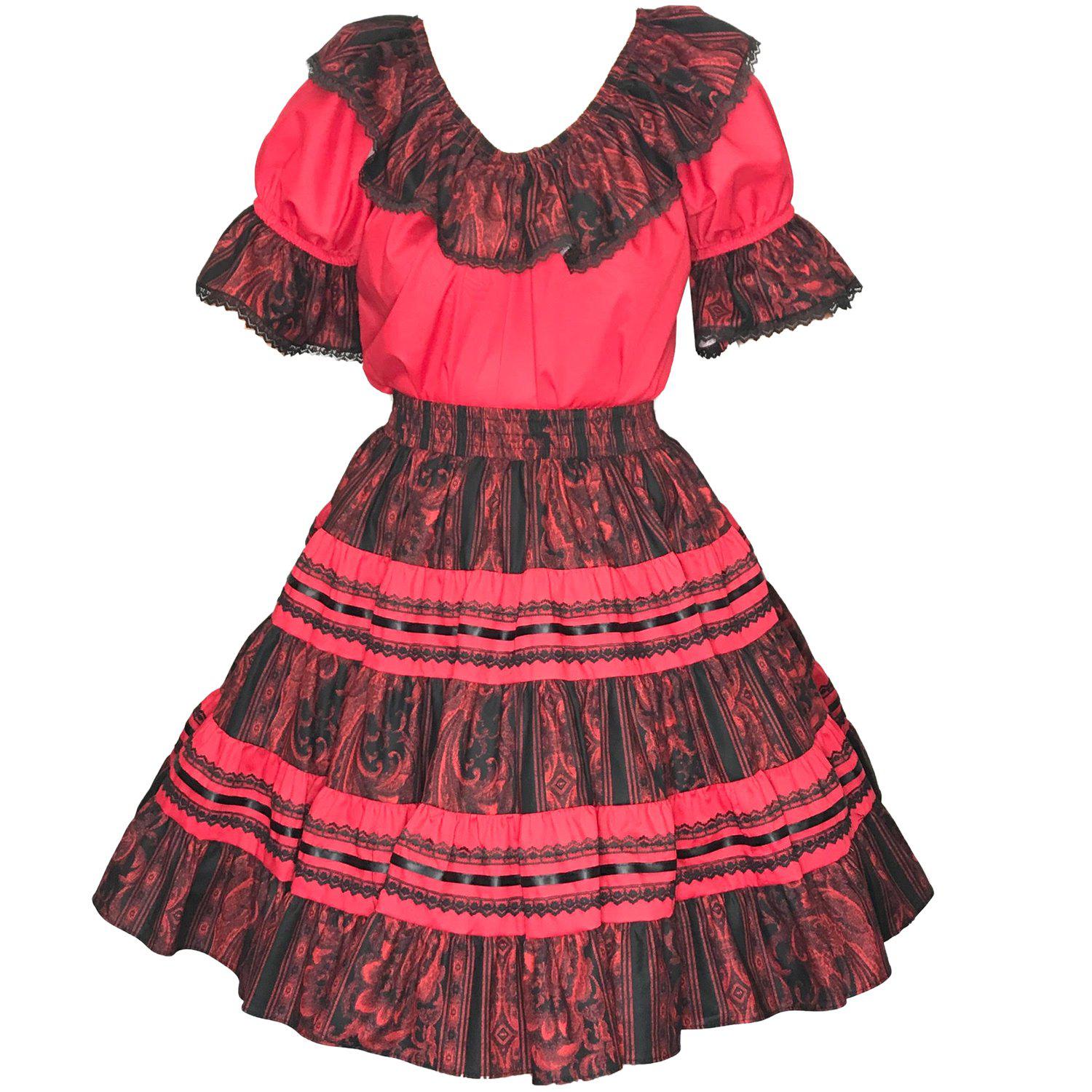This image features a professionally photographed, country-western themed dress suitable for a store's website. The dress presents a blend of rustic charm and formal elegance, with the bodice in a medium reddish-pink hue complemented by a delicate lace-trimmed Peter Pan collar. The short sleeves, edged with the same lace, radiate a quaint, nostalgic feel. Contrasting the bodice, a black overlay with intricate lace detailing extends down the dress. An elastic band at the waist, matching the lace pattern on the sleeves and collar, provides a snug fit, blending into a design landscape characterized by alternating reddish-pink and black lace bands. The skirt showcases an intricate, decorative arrangement of solid and striped bands, with the bottom third dominated by the dark maroon-black lace pattern, lending a sophisticated contrast to the otherwise vibrant attire. Overall, the dress appears diminutive, potentially tailored for a girl or petite woman, embodying a confluence of traditional flair and contemporary style.